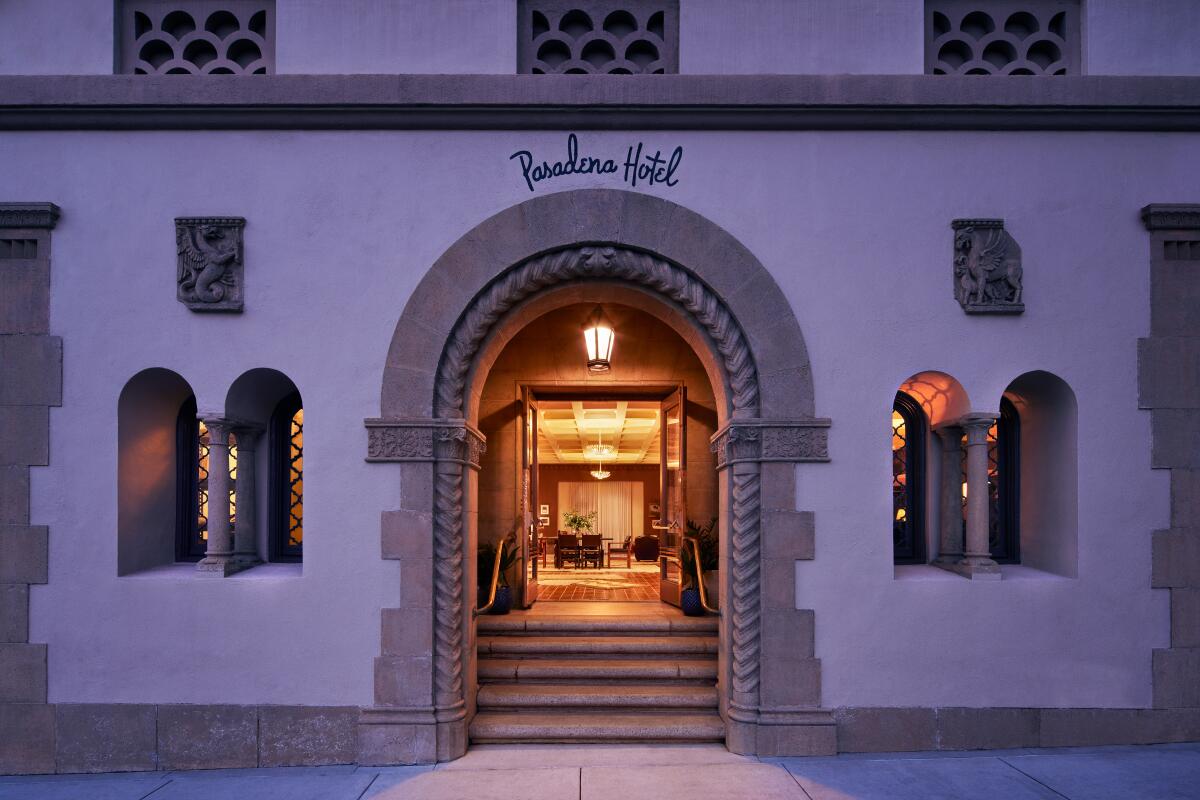This photograph captures the elegant façade of the Pasadena Hotel. The hotel's entrance features a grand archway constructed from a stone mix of gray and tan hues, adding a touch of classic charm. The front of the building is adorned in white stucco, further accented by additional patches of the same gray and tan stone. Above the archway, intricate black cursive lettering spells out "Pasadena Hotel." Flanking the windowsills are two small sculptures resembling mythical creatures or dragons, adding a whimsical touch to the architecture.

The entryway is reached via a set of inviting steps, leading to a large, open door that reveals a warmly lit lobby. Inside, a collection of comfortable brown chairs is arranged, awaiting visitors. The lobby's floor boasts a rich cherry wood color, contributing to the overall welcoming atmosphere of the space.